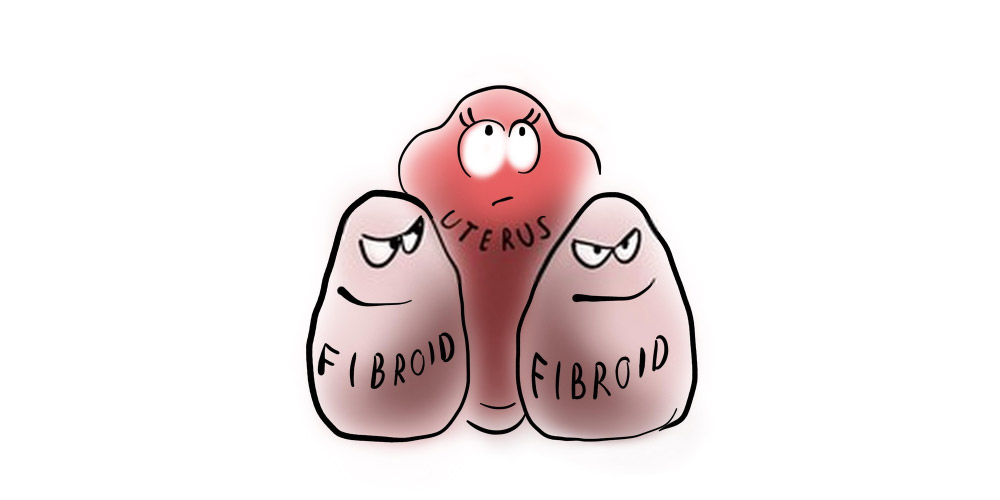The image is a cartoon depiction on a white background featuring three characters, illustrating a uterus and two fibroids. The fibroids are positioned on either side of the uterus, appearing smaller and menacing. Both fibroids have a potato-like or messy oval shape, with squinty, shifty eyes and mouths drawn as slashes or grins, giving them an angry and evil demeanor. The fibroids are colored in shades of brownish-gray, fading from darker to lighter. They each have "Fibroid" labeled across them in large black letters. 

In contrast, the uterus, centrally placed, is pinkish and shaped like a light bulb with subtle bulges. It has large, oval eyes adorned with eyelashes, conveying a more delicate and alarmed expression as if saying, "What do I do?" The uterus is also labeled in black letters below the character as "Uterus." The overall scene suggests the fibroids are closing in on the uterus, creating a sense of tension and discomfort.